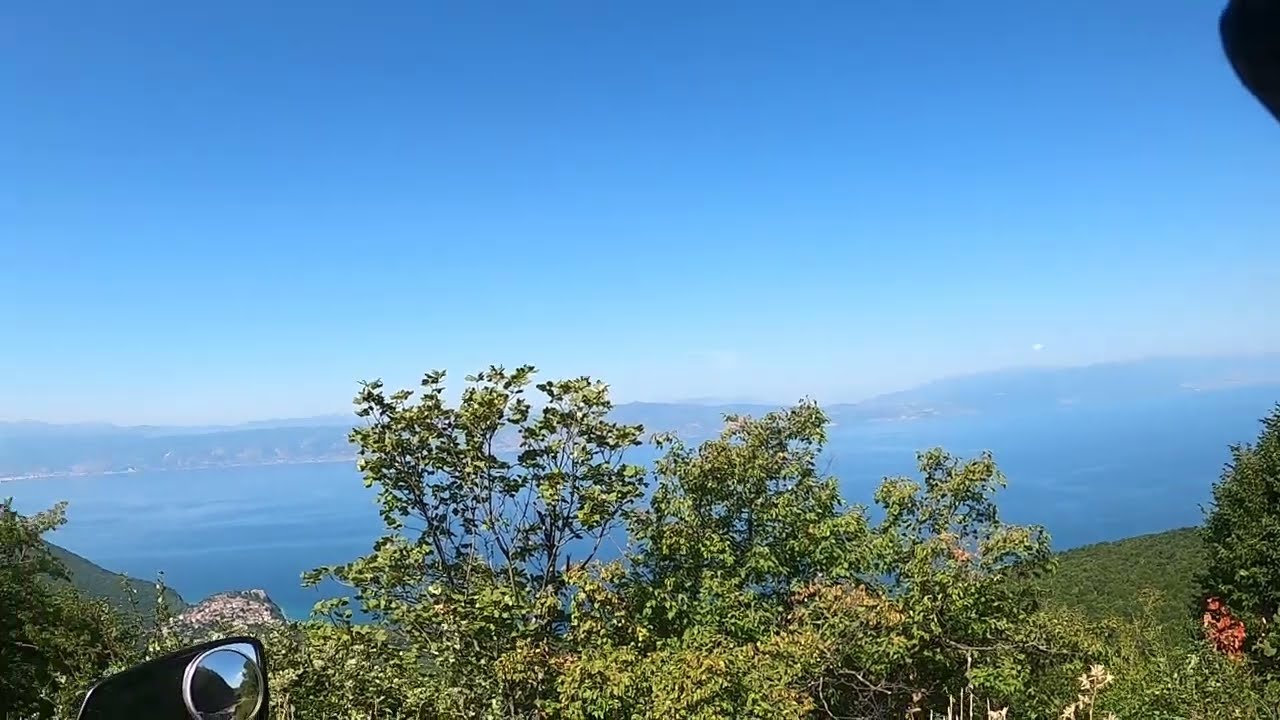The image captures a scenic view from the top of a hill, revealing a picturesque landscape. In the lower left-hand corner, the rearview mirror of a vehicle, possibly a car or motorcycle, suggests the image was taken from a parked vehicle. Dominating the scene are lush green trees and expansive bright green grass, with a hint of pink flowers on the lower right. A tree stands prominently beside a green hill. The middle of the image features the vibrant tops of trees with dense green foliage. On the horizon, a large, bright blue body of water stretches out, likely a lake, framed by rolling green hills and dotted with a distant cityscape. The clear blue sky, scattered with a layer of white clouds, completes the tranquil daytime setting. Behind the mirror, there appears to be a large rock formation, adding texture to the foreground. The overall composition masterfully combines the elements of land, water, and sky, enhancing the natural beauty of the scene.